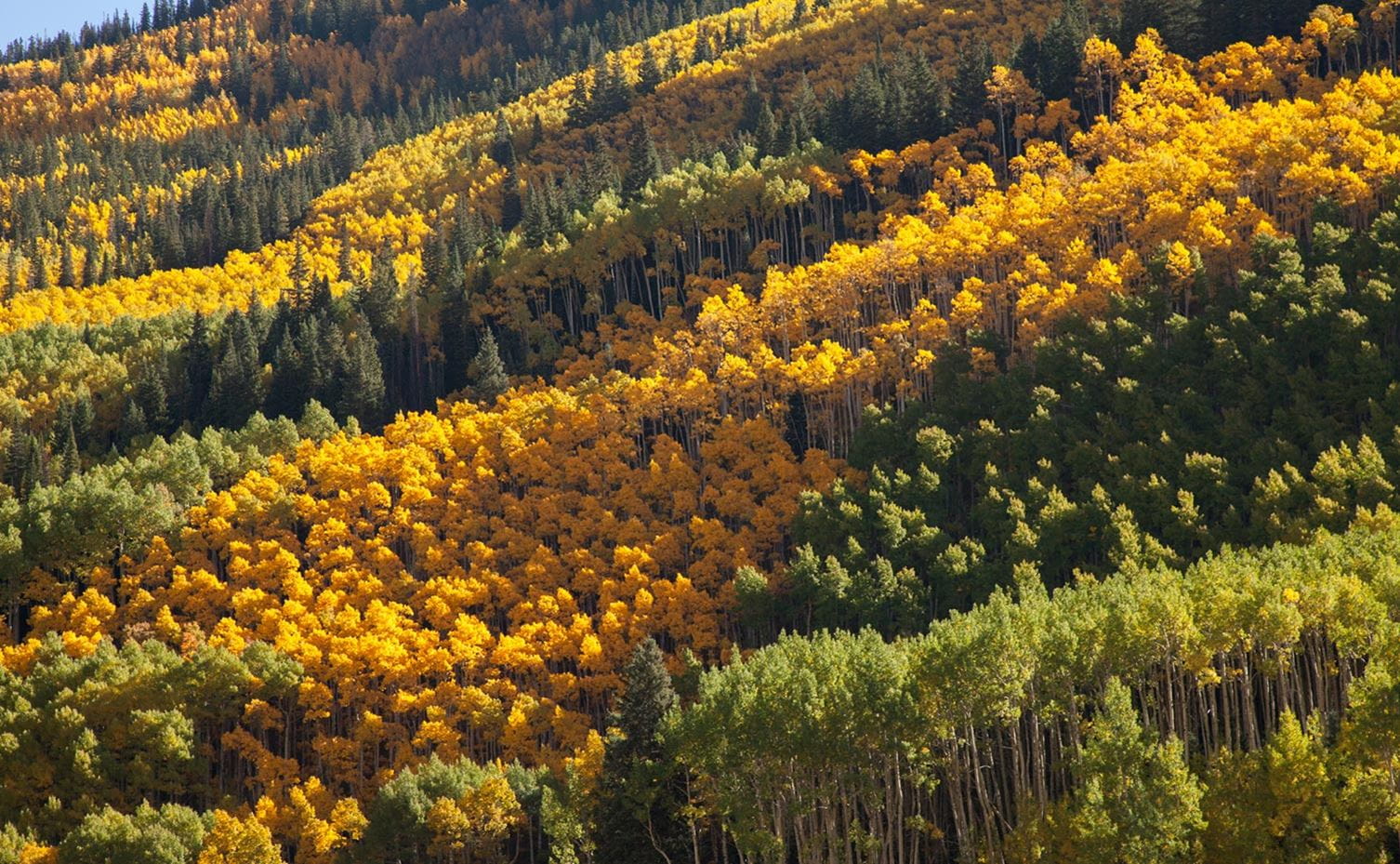This aerial photograph captures a breathtaking forest landscape during the fall season. The image, taken from a high vantage point, looks down on a diverse assortment of tree species. Half of the trees are in the midst of their autumn transformation, showcasing vibrant shades of orange and yellow, while the remaining trees retain their lush green foliage, including evergreen species. The trees are arranged in a somewhat organized pattern, suggesting a tree farm or a naturally layered forest on a hillside or mountain. The sunlight bathes the foliage in a warm glow, and patches of the clear blue sky peek through the tree canopy, highlighting the daytime setting. The meticulously arranged rows of trees, with varying foliage colors and sizes, create a stunning mosaic of nature's seasonal transition.